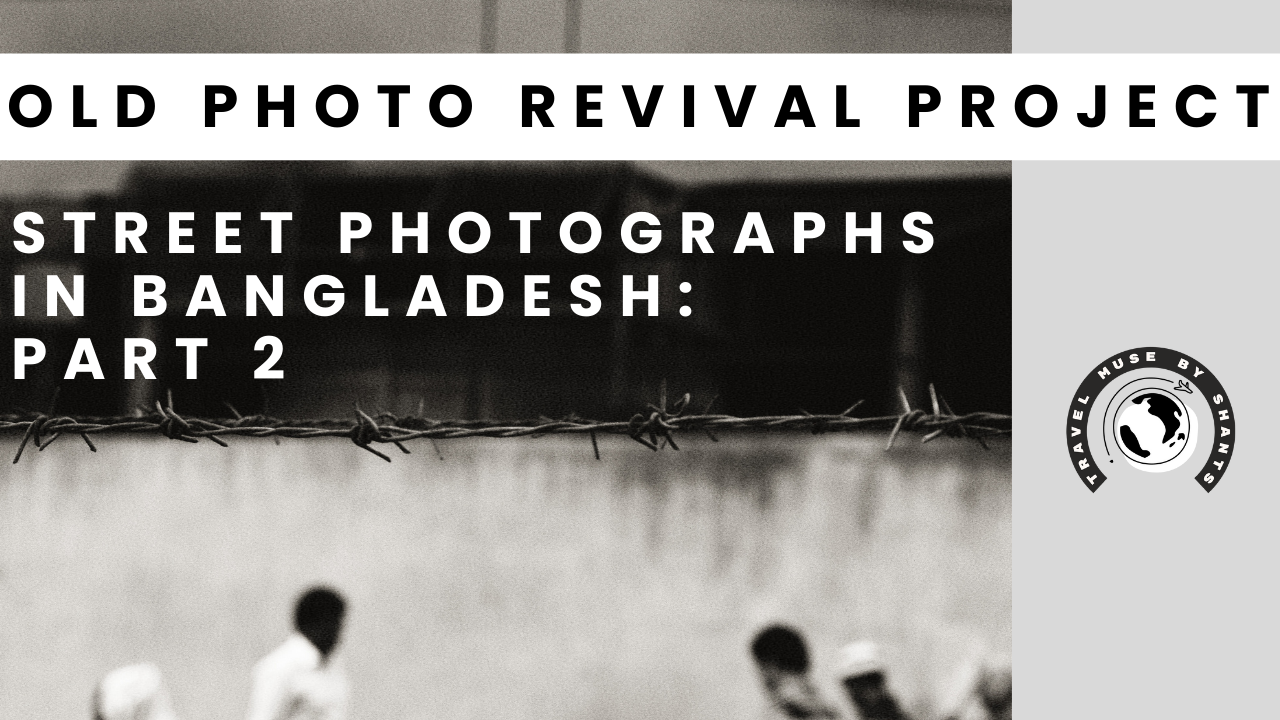The image is a black and white, monochromatic photograph with a blurred background that includes indistinct shapes of people's heads, a body of water, and a barbed wire spanning across the scene. The photograph is about one and a half to two times wider than it is tall, giving it a rectangular format. 

At the top of the image, a horizontal bar occupies the space from 5% to 15% down from the upper edge, serving as a header. This bar is gray and features black text that reads "OLD PHOTO REVIVAL PROJECT." Below this gray bar, aligned left in all capital white letters, the text continues with "STREET PHOTOGRAPHS IN BANGLADESH PART 2."

To the right side of the image, approximately in the center of the right-hand quarter, there is a logo against a solid gray background. This logo consists of a black circular border with white lettering around it, reading "Travel Muse by Chance." Inside this circular border, there is a white circle featuring a simple line drawing of the Earth with an airplane flying around it, representing travel themes.

In summary, the detailed caption would read:

"A monochromatic black and white photograph with a blurred background showing faint shapes of people's heads, a body of water, and a single barbed wire. At the top, a gray horizontal bar displays the text 'OLD PHOTO REVIVAL PROJECT' in black font. Below the bar, aligned left, white capital letters read 'STREET PHOTOGRAPHS IN BANGLADESH PART 2.' To the right, a gray area features a logo of a black circular border with 'Travel Muse by Chance' in white letters. Inside the circle, a simple line drawing of the Earth with an airplane flying around it completes the travel-themed logo."